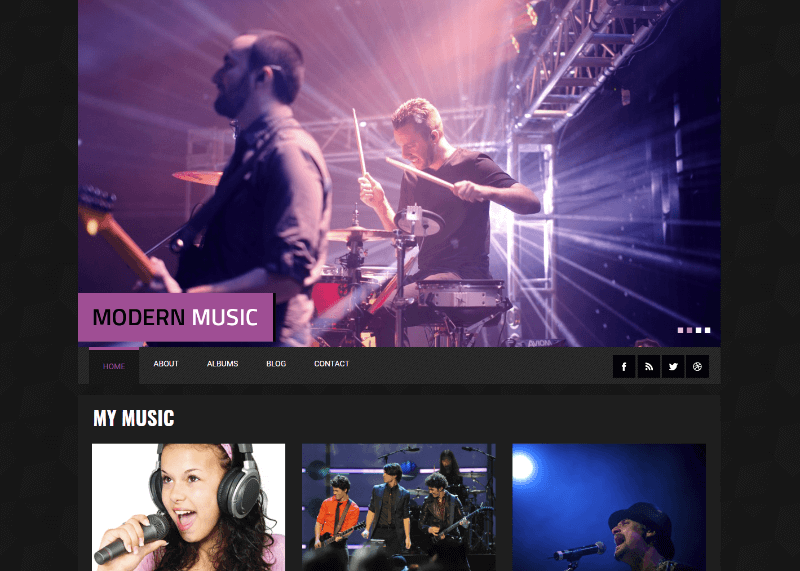A detailed caption for the provided image description:

---

**Screenshot of a Music Streaming Interface:**

The image presents a screenshot of a music streaming interface, set against a black background. The layout is slightly wider than it is tall. Occupying the top two-thirds of this interface is a vivid scene of a live concert. Central to this scene is a dynamic drummer, energetically playing his drums, with radiant stage lights illuminating him from behind, creating an electrifying atmosphere. 

To the left of the drummer, a guitarist can be seen, slightly turned to his left, adding depth to the concert setup captured in the image. Overlaying this concert scene, on the lower left section, is a small, purple rectangular banner with the text "Modern Music" in contrasting colors—'Modern' in black and 'Music' in white.

Directly beneath the concert scene, there is a row of navigation options, with the first one highlighted in purple (presumably indicating 'Home'), and the rest in white. Although some text is too small to decipher clearly, the last option in the row is labeled 'Contact'.

Towards the bottom right of the interface, below the picture, are three small icons, resembling the Facebook, Wi-Fi, and Tweet symbols, likely providing quick access to social features.

In the bottom section of the screenshot, the text "My Music" appears in white on the left side. Three image thumbnails are partially visible below this text, each portraying different musicians. The first thumbnail showcases a close-up of a woman singer with headphones and a microphone, the second shows a trio band, and the third features another artist singing into a microphone with a light source visible in the upper left corner of the thumbnail.

Overall, the interface exudes a modern vibe with its sharp contrasts, vibrant imagery, and user-friendly icons, capturing the essence of a robust music streaming experience.